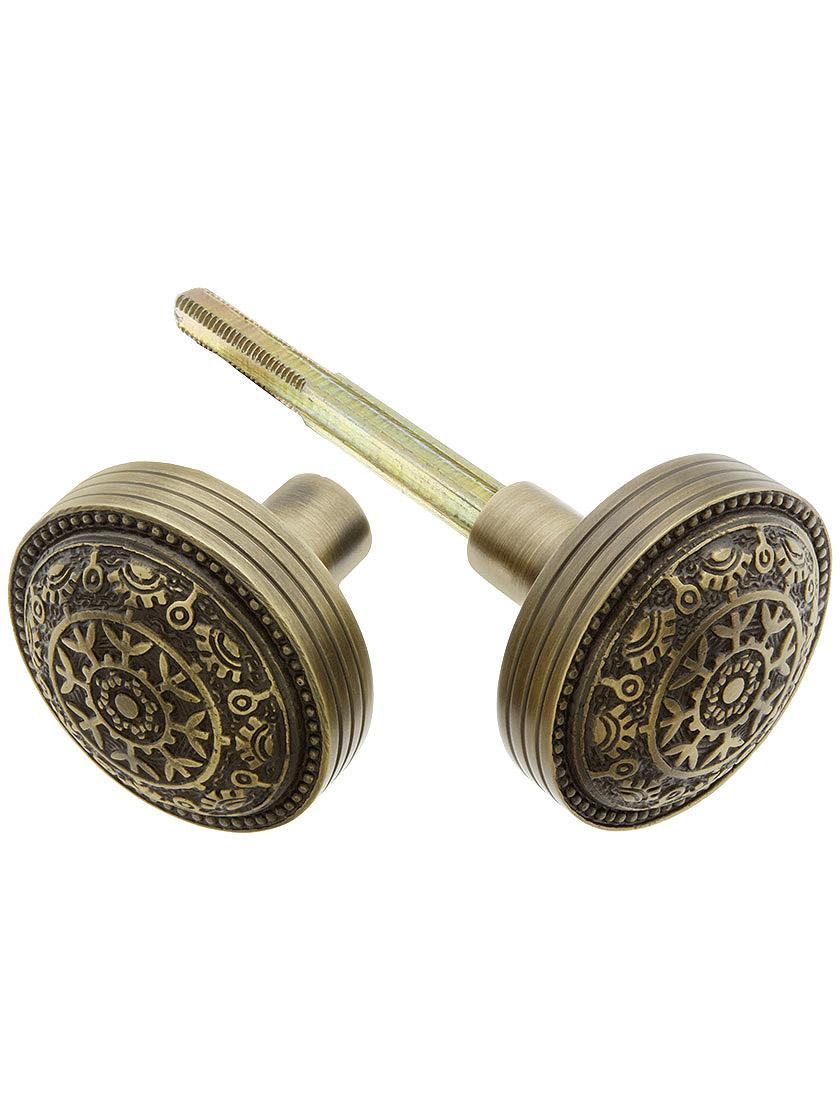This very close-up image features a pair of intricately designed cufflinks made of brass or a similar metal. The cufflinks are in two parts, with one piece unscrewed and situated to the bottom left and the main piece to the bottom right. The main part, resembling a circular head or cap, showcases a complex and ornate design. The center features a dot surrounded by a floral motif, followed by a snowflake pattern, a solid ring, and outer leafy patterns, all contributing to a clock gear-like aesthetic. The sides of the main piece display three grooves encircling the object. The part that screws in, which is slightly lighter and shinier, indicating a different or less tarnished metal, connects to a shaft tapering down with visible male threads at the end. This allows it to screw securely into the other part. Both pieces exhibit meticulous craftsmanship with their elaborate engravings and design. The background provides no contextual clues, merely a white expanse that emphasizes the detailed artistry of the cufflinks.